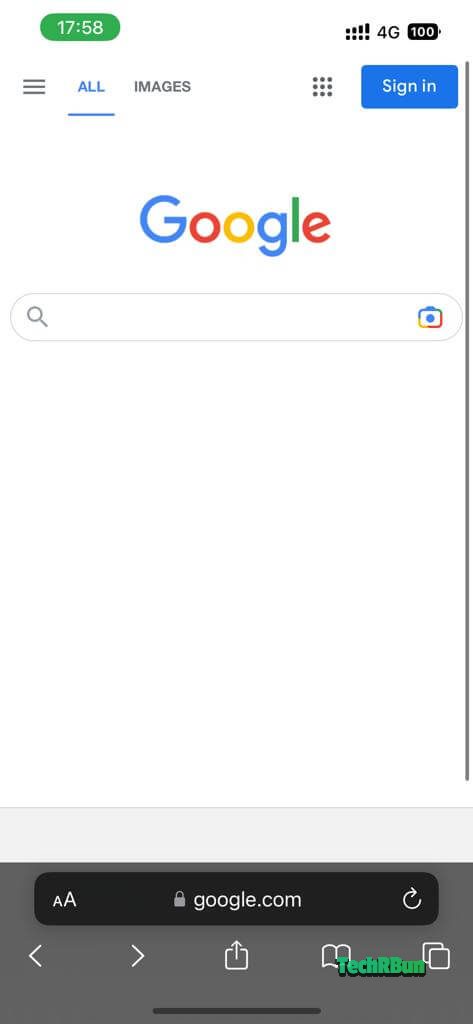The image showcases a minimalist scene of a user preparing to make a Google search. Dominating the center of the screen is the iconic Google logo in its vibrant colors accompanied by the familiar search bar. Above this, the user is prompted to sign in. Beneath the search bar and occupying the bottom portion of the screen, a wide gray navigation bar is visible. This navigation bar features various options such as "Back," "Forward," and "Read," as well as a darkened text field indicating "Google.com" which is shown as secured or locked. On the top right corner of the screen, the word "TECHR BUN" is prominently displayed in green with "TECH," "R," and "BUN" all capitalized, standing out against the rest of the interface. The top of the screen offers limited search options, only displaying the tabs "All" and "Images."